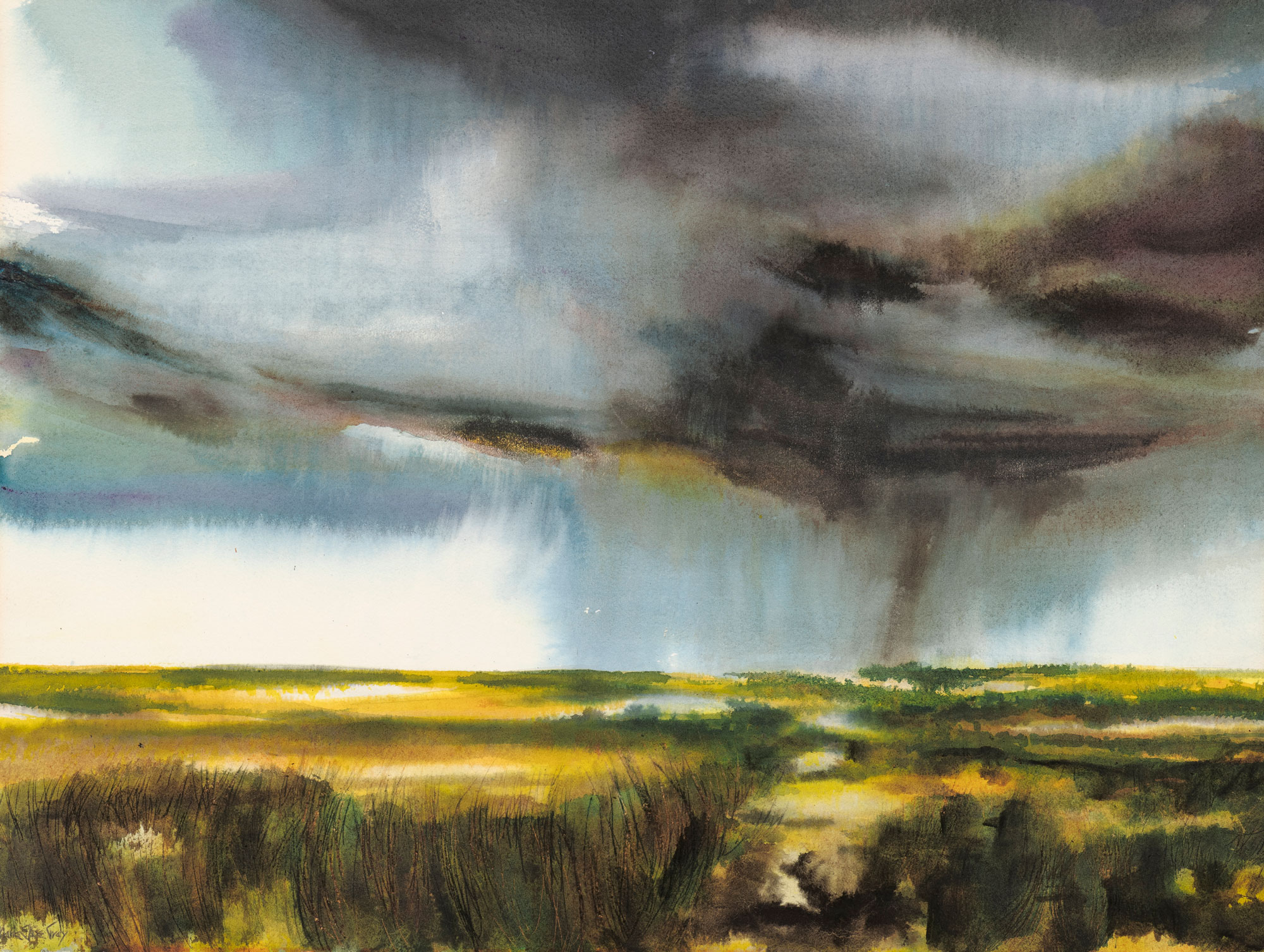The painting is a detailed, oil-like landscape of a field under a tumultuous sky. The lower portion features tall, lush grass in shades of dark green, olive, and yellow, interspersed with hints of black and patches of white, suggesting the presence of a small river or pond. Above the field, a stormy sky dominates the scene—with dark gray and black clouds swirling ominously. A well-defined funnel cloud on the right side indicates a forming tornado, set against an otherwise overcast sky. In the background, the horizon shows an eerie contrast of lighter white clouds, adding depth and highlighting the storm’s progression. No human structures or figures are present, emphasizing the raw, untamed beauty of the landscape.